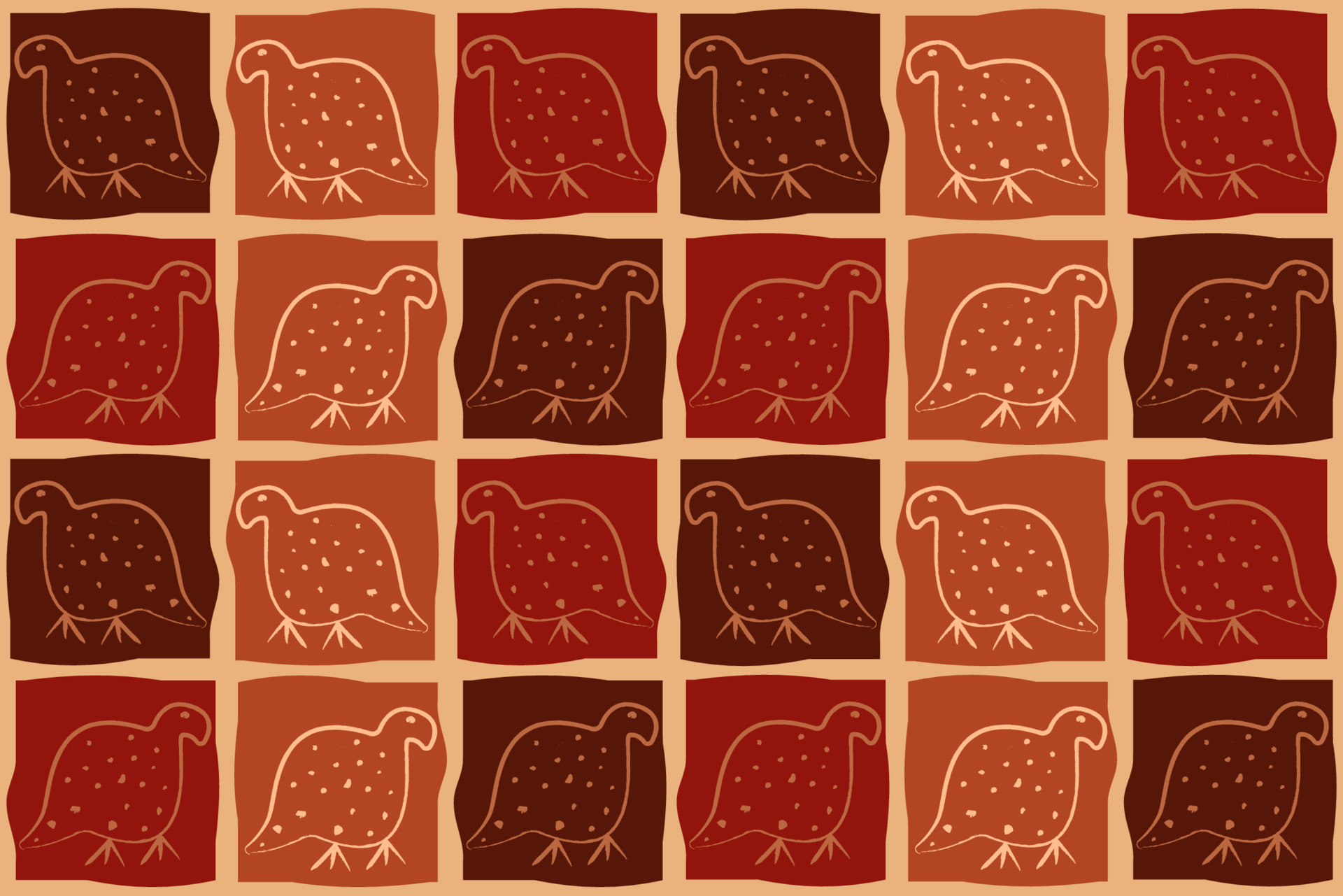The image is a quilted tapestry arranged in a 4x6 grid pattern, featuring stylized, crudely drawn birds embroidered in white outlines. Each bird has a round body, an oddly-shaped head resembling a semi-circle, a small tail without feathers, and two feet with three prongs. The birds are positioned in alternating directions; those in the top and third rows have their heads facing left and tails to the right, while those in the second and bottom rows face the opposite direction, with heads to the right and tails to the left. The squares in the grid vary in color in a rotating pattern, ranging from shades of brown and light brown to red and dark maroon. The bird designs also include speckled details scattered across their bodies.